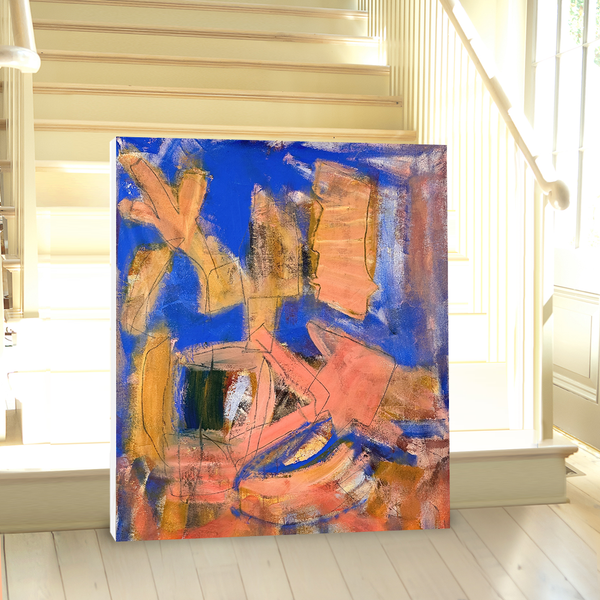The photograph, taken indoors on a sunny day, captures an artistic corner within a home featuring wood flooring and a prominent white staircase with white rails and balusters. Light from a window in the upper right section subtly illuminates the scene. The focal point of the image is a square abstract painting leaning against the staircase. This painting stands out with its primarily blue background and features an array of random brush strokes in brown, black, orange, and yellow hues. The artistic chaos of the piece does not form any recognizable shapes, but rather presents an intriguing mixture of brush strokes that resemble an X, rectangles, and random sideway lines. The sunlight hitting the painting adds a subtle glow, enhancing its vibrant colors.